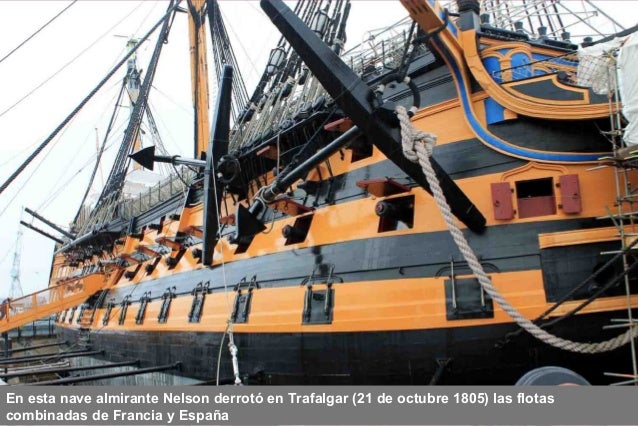The image depicts a remarkably detailed side view of a large, historic wooden battleship from either the 1700s or 1800s, potentially a replica of such a ship. The vessel, decorated predominantly with shades of black and orange-stained wood, features several distinctive elements. There are multiple rows of cannons visible through port windows along its side, with some of the cannon ports currently open. Notably, blue and yellow ornamentation embellishes the upper front section of the ship, complemented by intricate rigging of ropes ascending a series of tall masts which would support the ship's numerous sails.

The ship is currently on stilts in a dry dock, indicating that it is not in water. Various features such as black anchors, a yellow staircase leading to the center of the ship, and a ladder with an individual climbing it, add to the complexity of the scene. An informational graphic in Spanish at the bottom of the image includes a significant date: October 21, 1805. This date suggests a historical context, possibly linking the ship to Admiral Nelson and the Battle of Trafalgar. The outdoor setting, likely a marina, adds a sense of authenticity and historical ambiance to the scene.